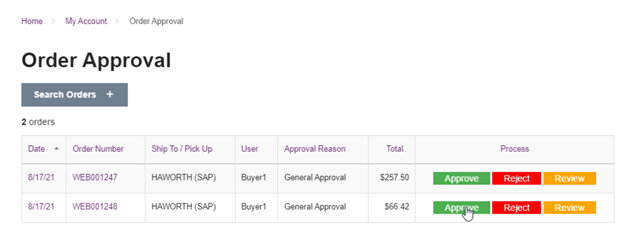The image features a clean white background. At the top, there are three blue buttons labeled "Home," "My Account," and "Order Approval." Below, a gray button titled "Search Orders" is visible. The main section displays two orders atop a light blue background. Each order entry includes the date, order number, shipping or pickup details, user, approval status, reason, total amount, and process options.

The first order, dated 8-17-21, shows order number WEB0001247 for "Hayworth SAP," requested by "Buyer 1," under "General Approval" status with a total of $257.50. For this order, there are three actionable buttons: a green "Approve" button, a red "Reject" button, and a yellow "Review" button.

The second order, also dated 8-17-21, shows order number WEB0001248 for "Hallworth SAP," requested by "Buyer 1," similarly under "General Approval" status with a total of $66.42. This entry has the same three actionable buttons for approval, rejection, and review.

A notable visual detail is a small hand icon positioned to click the green "Approve" button on the second order.